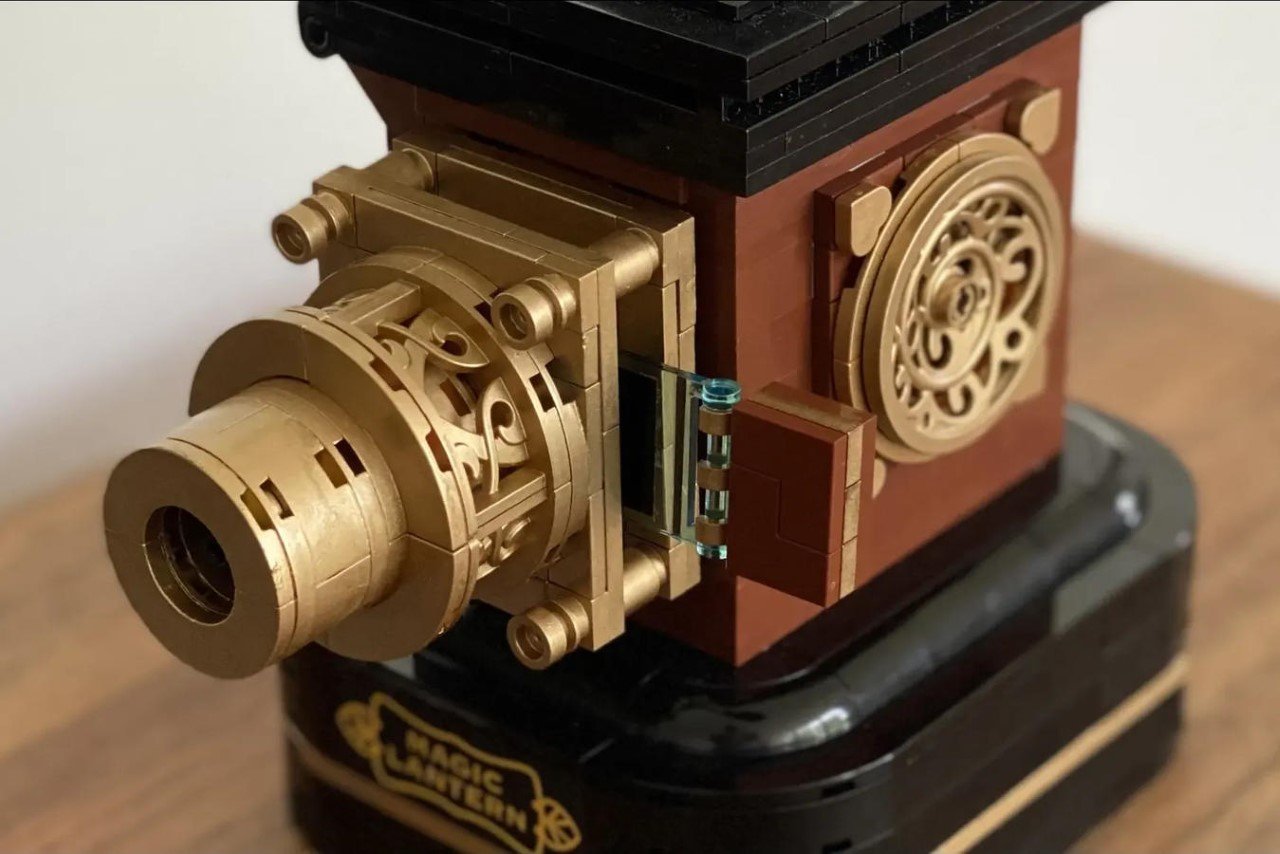This is a professional photograph showcasing a meticulously crafted reproduction vintage projector made entirely out of Lego pieces. The Lego projector, embellished in rich colors of black, brown, and gold, showcases intricate details with a striking visual resemblance to an antique Magic Lantern projector. The projector is seated prominently on a wooden table against a stark white wall backdrop, highlighting its vibrant construction. 

The sturdy black base of the projector features a prominent gold stripe and bears the "MAGIC LANTERN" logo in elegant gold font. The main body of the projector, constructed from brown Lego pieces, forms a cohesive unit as the diverse blocks stack neatly together. Distinctive golden Lego pieces form the lens casing at the front, imparting a sense of ornamental grandeur. Additionally, a large, round decorative piece, resembling floral filigree, adorns the side, adding to its vintage charm.

The top of the projector is accented with more black Lego pieces, finely assembled to complete the retro aesthetic. This close-up view allows for appreciation of the craftsmanship and detailed assembly, making the Lego reproduction both a nostalgic homage and a notable work of art.